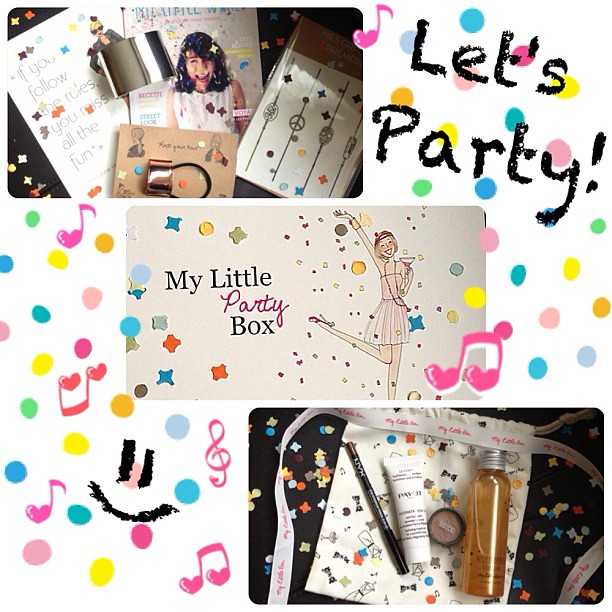This is a large square graphic with a vibrant, confetti-like theme. The background is white, adorned with colorful polka dots and musical notes that feature heart shapes instead of traditional note heads. In the upper right-hand corner, in a playful black crayon-like font, the text reads, "Let's party!"

In the upper left section, there is a rectangular image resembling a magazine cover, showcasing a young girl surrounded by scattered items, embodying the saying "If you follow the rules you miss all the fun." This image has a whimsical and carefree vibe, enhanced by an adjacent sheet decorated with dots, stars, and peace signs.

The middle section highlights a rectangular outline illustration of a girl in a small summer dress, striking a playful pose with a wine glass in hand, dancing amidst confetti. This represents the packaging design for "My Little Party Box."

In the lower right section, there is a display of beauty and self-care products, including lip gloss, eyeliner, a white lotion tube, a round makeup case, and a bottle with gold liquid. These items rest atop a canvas pull-string bag, with confetti scattered around, contributing to the festive atmosphere.

Overall, the graphic blends elements of celebration and self-care, underscored by the colorful polka dots, musical notes with heart shapes, and the inviting message, "Let's party!"